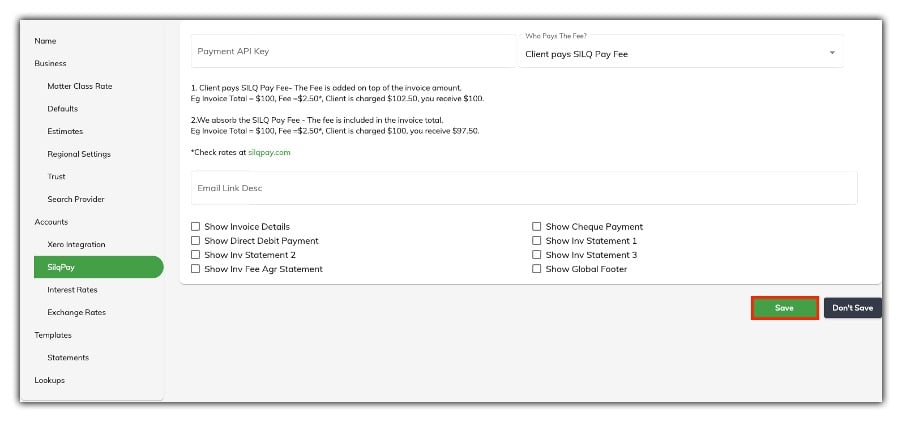A comprehensive screenshot of a web page showcases a detailed user interface for managing business settings and payment configurations. On the left side of the screen, a vertical menu features several options: Name, Business, Master Class Rate, Defaults, Estimates, Regional Settings, Trust, Search Provider, Accounts, and Zero Integration. Further down, the menu includes another set of options displayed in a green tab: SLQ Pay, Interest Rates, Exchange Rates, Templates, Statements, and Lookups.

In the main content area to the right, the focal point of the web page is a section labeled "Payment API Key," which handles the fee payment settings. A dropdown menu is selected to show "Client Pays SLQ Pay Fee." Detailed textual information elaborates that the client pays the SLQ Pay fee, illustrating this with an example: If the invoice total is $100 and the fee is $2.50, the client will be charged $102.50, and the business will receive $100.

At the bottom of the page, a prominent green button outlined in red displays the text "Save," accompanied by a black button labeled "Don't Save." The layout and color coding facilitate user interaction, ensuring clarity in executing commands related to payment and invoice settings.